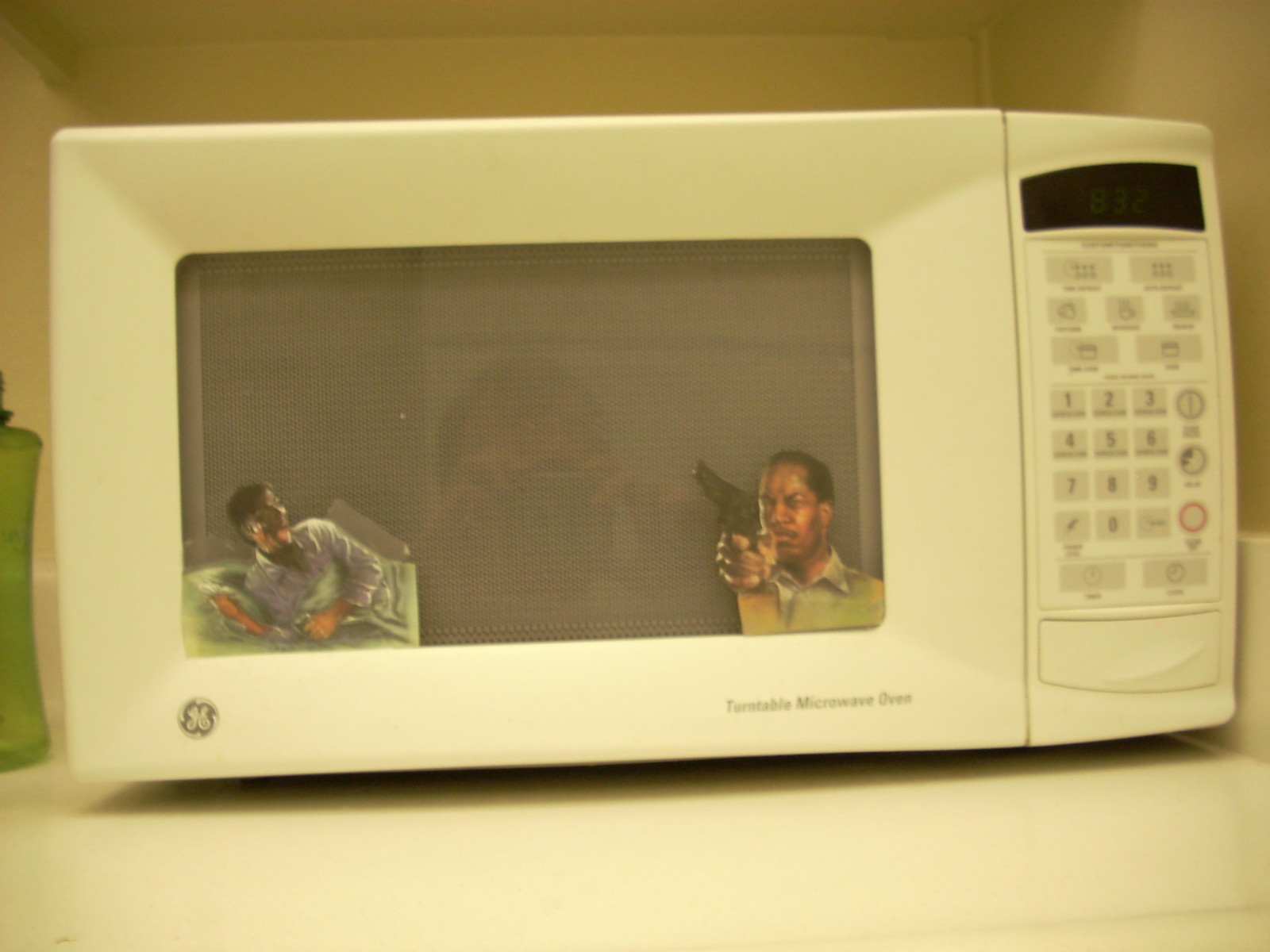The image features a white GE Turntable Microwave Oven set against a beige wall and positioned in the corner of a white kitchen counter. The microwave displays a familiar array of buttons and a digital interface on the right side, including the clock reading 8:32 in green text on a black background. The GE logo is visible on the lower left corner, and the phrase "Turntable Microwave Oven" is written on the lower right. Notably, the microwave is unplugged. 

On the microwave's door, two stickers are prominently placed: one on the left side depicts a black man resembling Michael Jackson in the "Thriller" music video, appearing startled in bed with green sheets and white pajamas. The sticker on the right corner shows another black man squinting and holding a gun, finger on the trigger, and dressed in a greenish-yellow collared shirt. 

In the reflection on the microwave's panel, a male-presenting individual with short hair is seen taking the photo using what seems to be a digital camera, with a refrigerator faintly visible behind him. To the left of the microwave, partially out of the frame, there is a green object that might be a vase or water bottle.